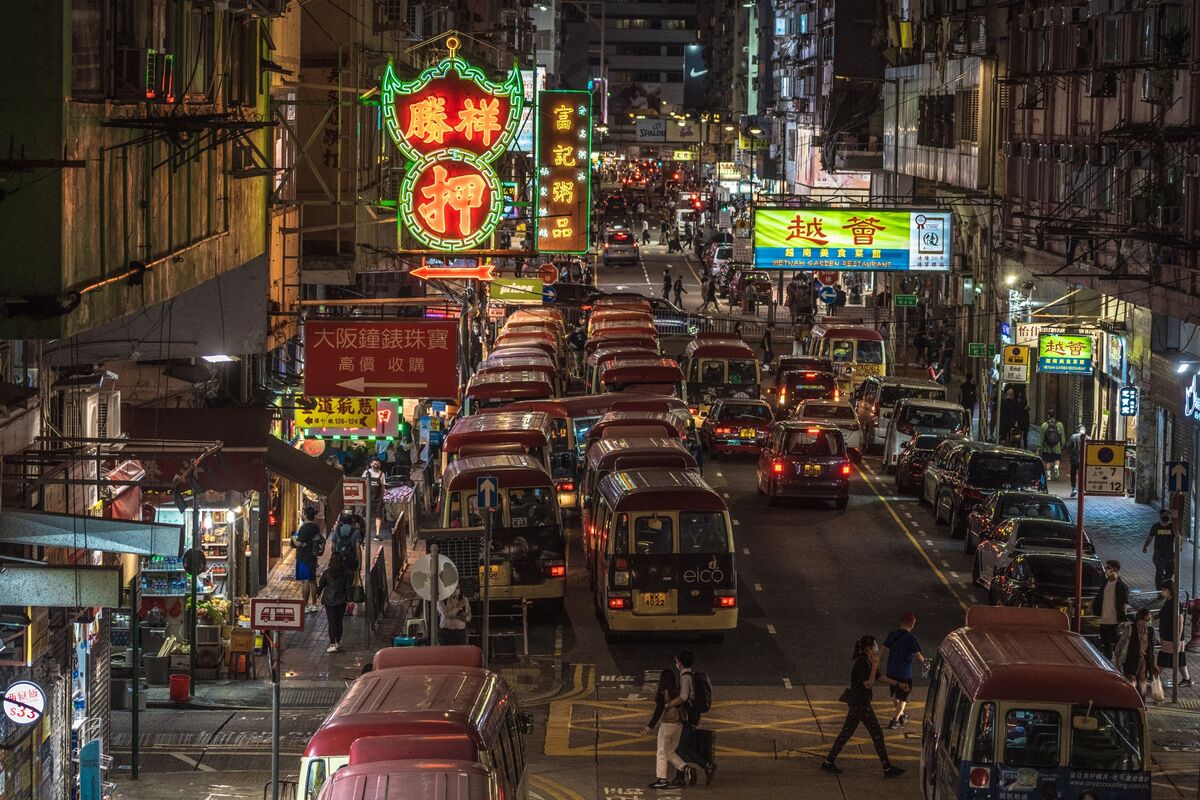The image features a bustling downtown area of an Asian city at night, likely in Japan or China, given the illuminated signs adorned with Japanese or Chinese text. The vibrant scene is characterized by a multitude of colorful neon signs in hues of green, gold, maroon, blue, and red, which advertise various shops and eateries lining both sides of a busy street. Numerous identical small vans with red tops and yellow bodies occupy half of the roadway on the left side. The scene extends into the distance, suggesting a large urban environment. Pedestrians can be seen using crosswalks and walking along the sidewalks. The urban landscape is dotted with high-rises, adding to the sense of a densely packed city. Among the lit signs, some notable ones include a neon green outline with bright orange characters and a horizontal sign featuring green with red characters. The nighttime ambiance is accentuated by the glow of taillights from cars and buses, adding to the dynamic atmosphere of the city street.